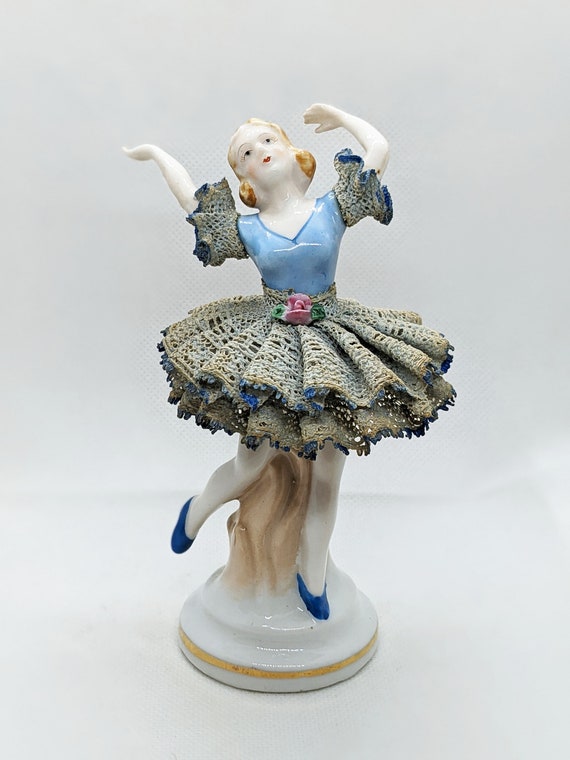This image features a highly detailed ceramic figurine of a ballerina, showcased on a white circular base with a delicate gold border. The ballerina is mid-dance, her arms gracefully raised above her head, emphasizing her fluid movement. She wears a light blue blouse adorned with matching ruffled sleeves that extend to her elbows. Her skirt, a layered ruffle affair, flows around her, predominantly white with subtle black and green accents, giving an impression of gentle motion. She has finely painted dark blue shoes that contrast with her otherwise porcelain-white appearance.

The figurine's blonde hair is meticulously sculpted and painted, adding to the lifelike quality of her features, including two dot eyes and red lips. The base also includes a small piece of what appears to be a textured representation of wood, possibly part of a tree, behind her. This striking piece stands approximately six to eight inches tall, capturing the essence of a dancer in the midst of a poised and elegant ballet performance.